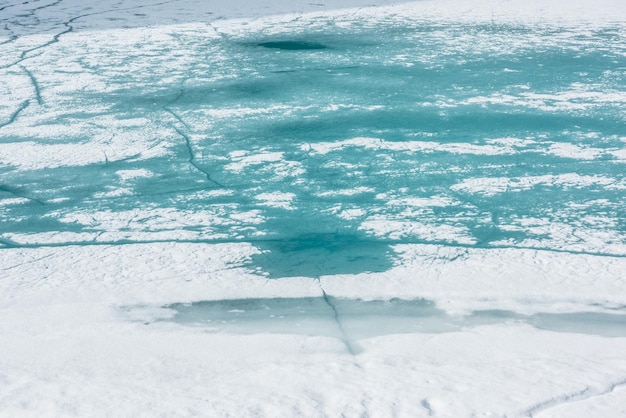The image captures a close-up view of a thin layer of snow partially covering a sheet of ice. The ice beneath the snow has a distinctive greenish-blue hue, while the snow is scattered and cracked, revealing the surface below. In the upper left and top sections, the snow appears as faint, white lines atop the ice. Towards the lower center, a small, darker teal pool of liquid is visible, suggesting uneven melting. This pool stands out against the predominantly greenish-blue ice and a thin snow cover that isn't very deep, sparsely covering the ground. There are several cracks and lines present both beneath and upon the snow, adding texture to the scene. Overall, the photograph distinctly captures the nuanced transitions between the melting snow and the colored ice beneath it.